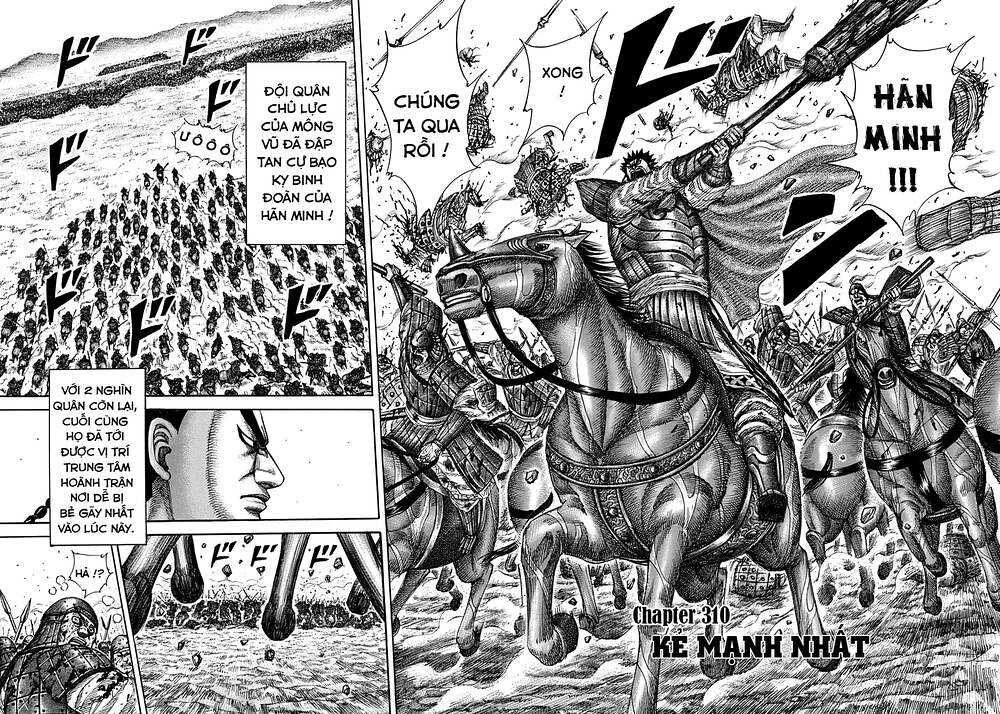The black and white detailed caricature drawing appears to be a page from a comic book or manga, potentially Vietnamese or Thai. The artwork is divided into five sections, with intricate, finely penciled details and text in a foreign language. The largest section on the right depicts a chaotic war scene with numerous soldiers on horseback charging from right to left, wielding weapons, and causing destruction, with figures flying through the air. Above this, a smaller section shows an overhead view of the frantic battle, accompanied by explanatory text in foreign lettering.

On the left side of the page, the top block frames a group of men on horses, arranged in a triangular formation, moving towards a gate. Beneath this, a narrow section highlights a close-up profile of an angry man, his eyebrows knit in fury as he glares to the left. The bottom left block features a soldier clad in armor looking back with a puzzled expression, and the final block to the right of it captures the hooves of running horses. At the bottom of the page, the text "chapter 310, K-E-N-A-N-H, N-H-A-T" is written, anchoring the elaborate scene of wartime tumult and intense emotions.